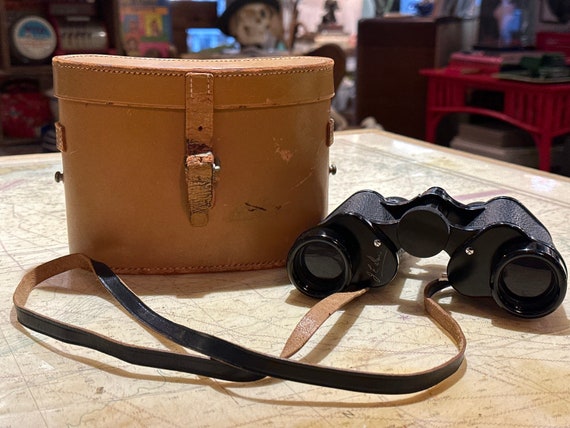This detailed color photograph captures a pair of classic black binoculars next to their vintage light brown leather case, both resting on a cream-colored tabletop. The binoculars feature a distinctive strap that is black on one side and tan on the other. The case, with its buckled strap and additional leather and brass attachments on either side, appears well-worn and slightly discolored, suggesting significant use over time. Intricately stitched, the case has a belt-loop strap that secures through a silver buckle. The background of the image hints at an eclectic or antique store setting, featuring a variety of peculiar objects such as a red desk, a brown bureau, and a highly stylized, grinning Day of the Dead skeleton head in black and white. The composition and elements suggest a scene rich in history and character, offering a glimpse into a space adorned with unique, timeless artefacts.